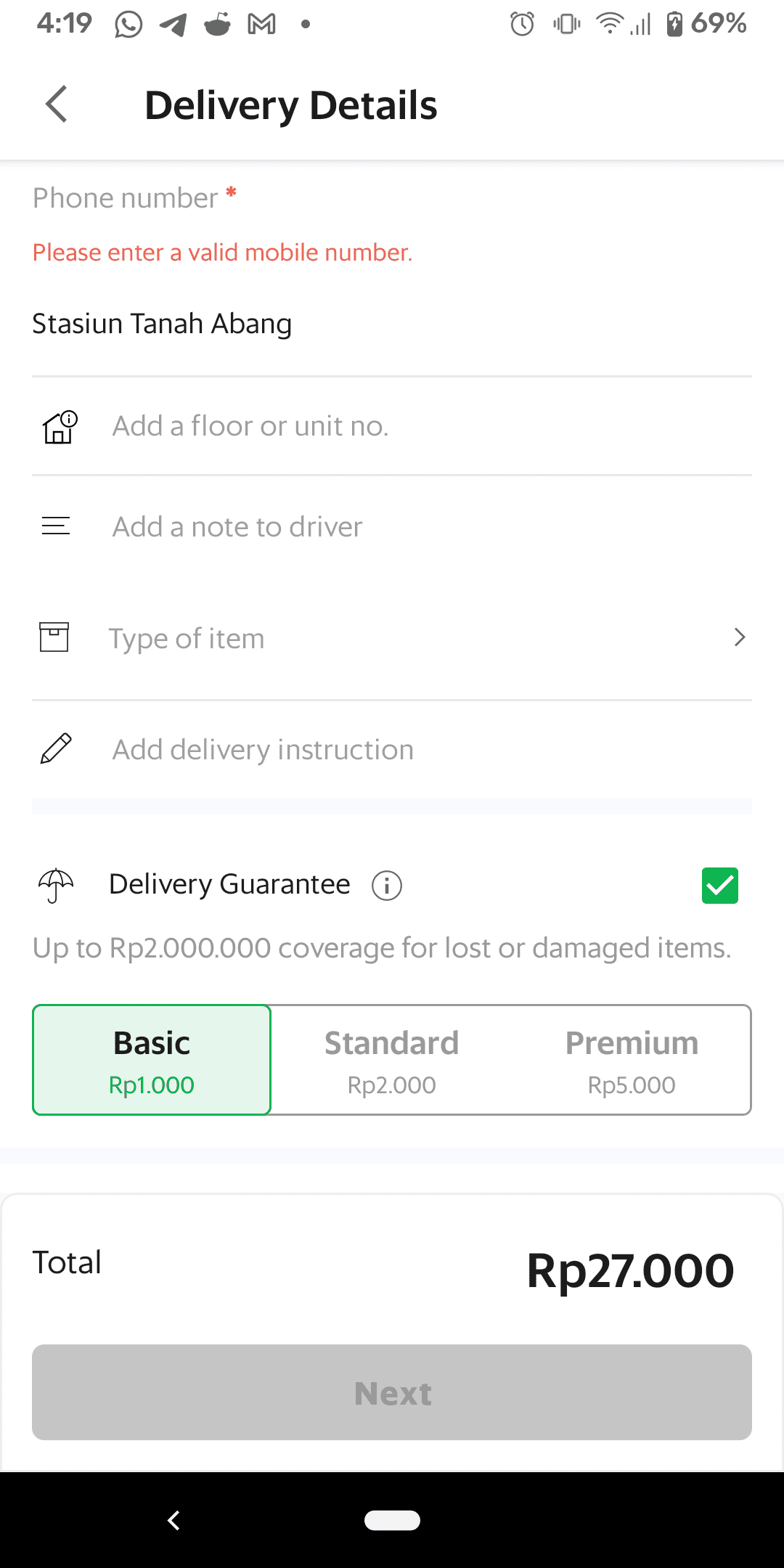A mobile phone screenshot of a shopping page is displayed, featuring prominent black text on a white background. At the top of the screen, delivery details are visible, hinting at the nature of the page. Above these details, the user interface displays the status bar with "4:19" on the left, followed by icons for signal strength, Wi-Fi connection, battery status at 69%, a Reddit icon, a clock icon, and a mobile phone icon. 

Directly beneath this, the delivery details heading appears, accompanied by a back arrow. Below it, a phone number field is shown with an error message in red, "Please enter a valid phone number," and miswritten as "Tara Abang," which is clearly not a phone number. 

Further down is a house icon prompting for additional information such as the floor or unit number, followed by fields to add notes, specify the type of item, and provide delivery instructions. 

A section featuring a green tick-box labeled "Delivery Guarantee" is visible next, ensuring coverage up to RP23000000 for lost or damaged items. Multiple delivery options are listed with costs: Basic (RP1000, ticked on the left), Standard (RP3000), and Premium (RP5000). 

The total amount due is RP27000, displayed at the bottom-right corner of the screen, just above a gray "Next" button. A black navigation bar at the bottom features a small, white, curved rectangle in the center with a back arrow pointing left.